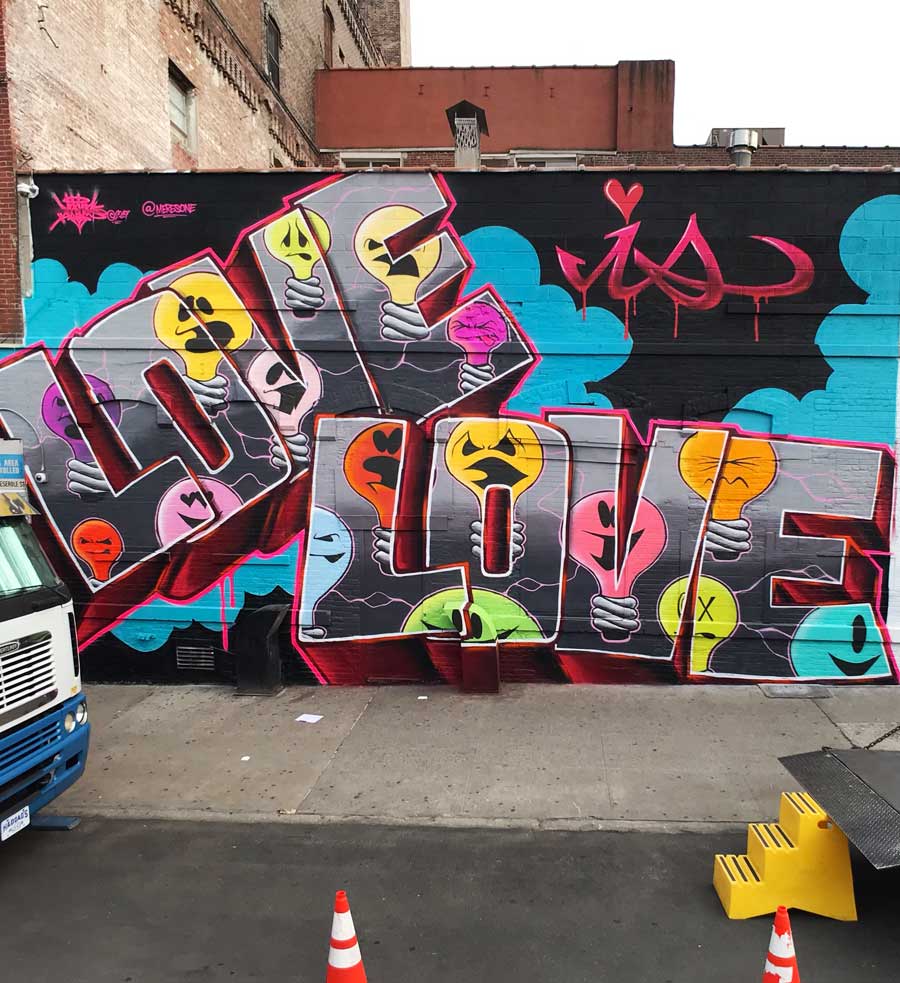This detailed photograph captures a street view of a vibrant mural adorning the exterior wall of a brick building in a city. The scene is captured from an elevated level, providing a downward perspective on the dark gray street below and the light gray sidewalk running parallel to the building. On the far left side of the image, the front end of a white and blue truck or bus is visible. 

Dominating the middle section of the frame, the mural features the word "LOVE" twice: once diagonally in large blocky letters at an upward angle, and again horizontally at the bottom. Each letter is creatively filled with colorful, animated light bulb characters exhibiting various facial expressions. These whimsical light bulbs are in shades of yellow, orange, pink, red, purple, and have X's over some of their eyes, contributing to an array of emotions from happy to sad, and scared to angry.

The mural's background is predominantly black, adorned with playful blue clouds and pink areas. To the left, the word "IS" with a heart-dotting the "I" and a small logo nearby add further detail to the mural's message. The overall ambiance suggests an overcast day, with a gray sky overhead and additional red brick buildings visible in the background. Orange traffic cones are spotted on the sidewalk, enhancing the urban street setting of this creatively expressive and detailed mural in the heart of the city.